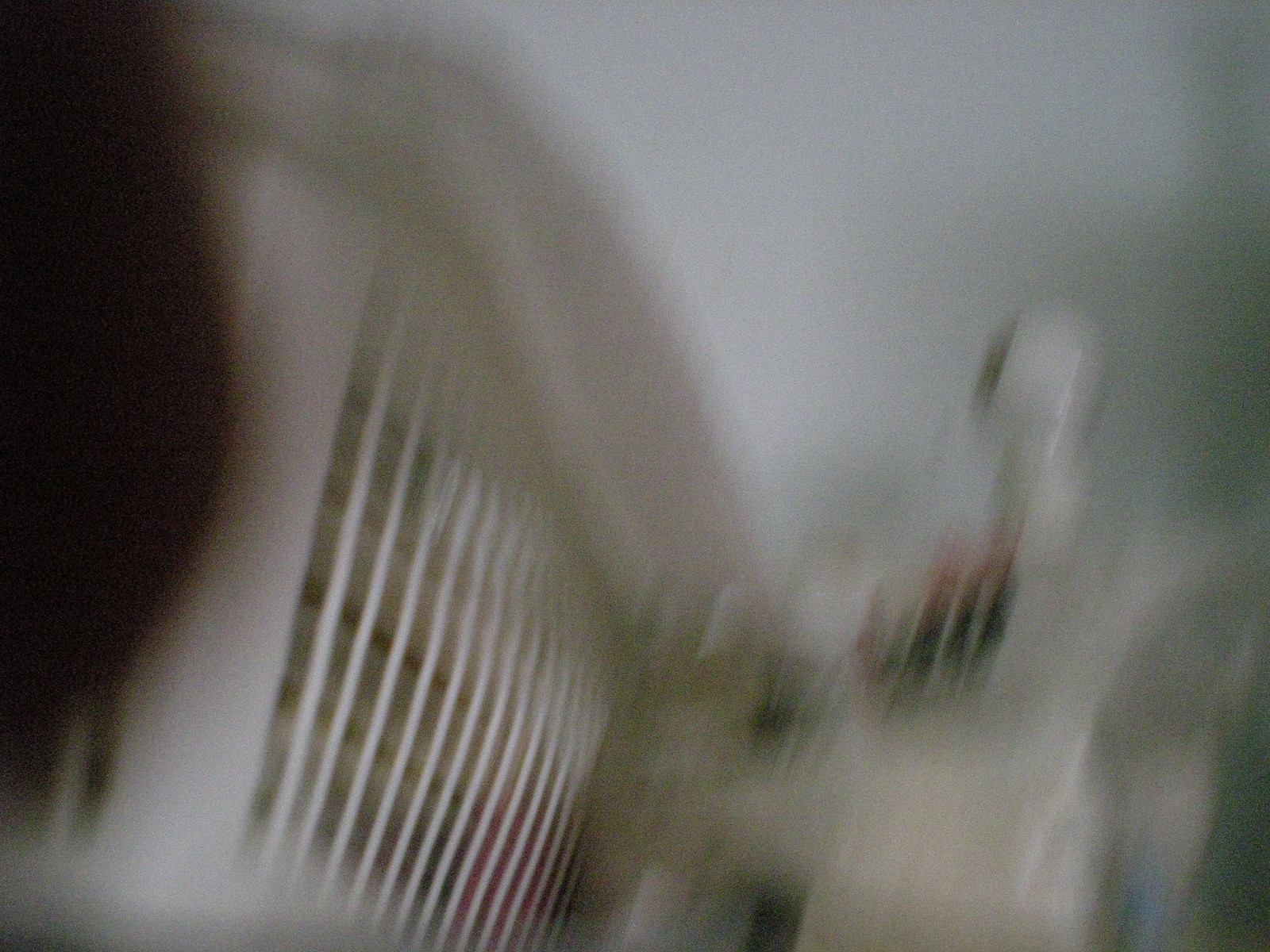The image is rectangular and approximately 20% wider than it is tall, with significant blurriness as if the camera was jolted while capturing the scene. Dominating the left side of the photograph, occupying almost 50% of the frame, is an upside-down white laundry basket with vertical, off-white slats. Just to the left of the basket, there appears to be a dark brown, possibly reddish object, which looks like hair. To the right of the basket, a humanoid-like figure with a white head, black visor, white neck, and chest can be observed, although the blurriness makes its identity ambiguous. There are shadows cast beneath the laundry basket and alongside the other objects. The background includes an off-white ceiling and a white wall, with additional shadows creating a darker shade in the upper right corner of the image.